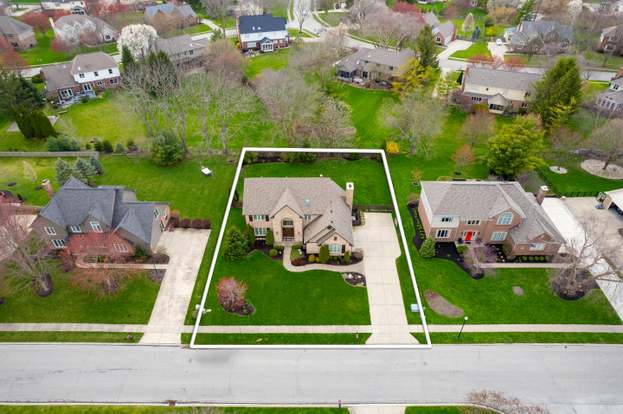This image provides an overhead view of a well-manicured upper middle-class neighborhood, captured as if from a drone, showing a layout suggestive of a housing development. The focal point of the image is the house positioned centrally at the bottom, distinguishable by a white rectangular outline around it, highlighting the property boundaries. This featured house has a light brown brick exterior, two stories, a large driveway situated on its right side, and well-maintained green lawns in both the front and back yards adorned with a few small trees and bushes.

In the immediate vicinity, there are two other houses lined up along the bottom of the image, flanking the highlighted house. The house on the left has a pointy roof and brown frontage with two trees in its front yard, while the house on the right features light brown brickwork and a single tree. Each of these houses also boasts two floors and sizable green lawns. 

Above these three houses, the image reveals additional homes arranged closely together, typical of a neighborhood development. The further back from the focal house, more homes appear partially visible, numbering around ten in total, with four noticeably small houses in the far right corner and several others with features like large gardens and two floors. Grey roads and sidewalks connect the houses, with the main street running along the bottom of the image, accentuating the structured and interconnected nature of this residential area.